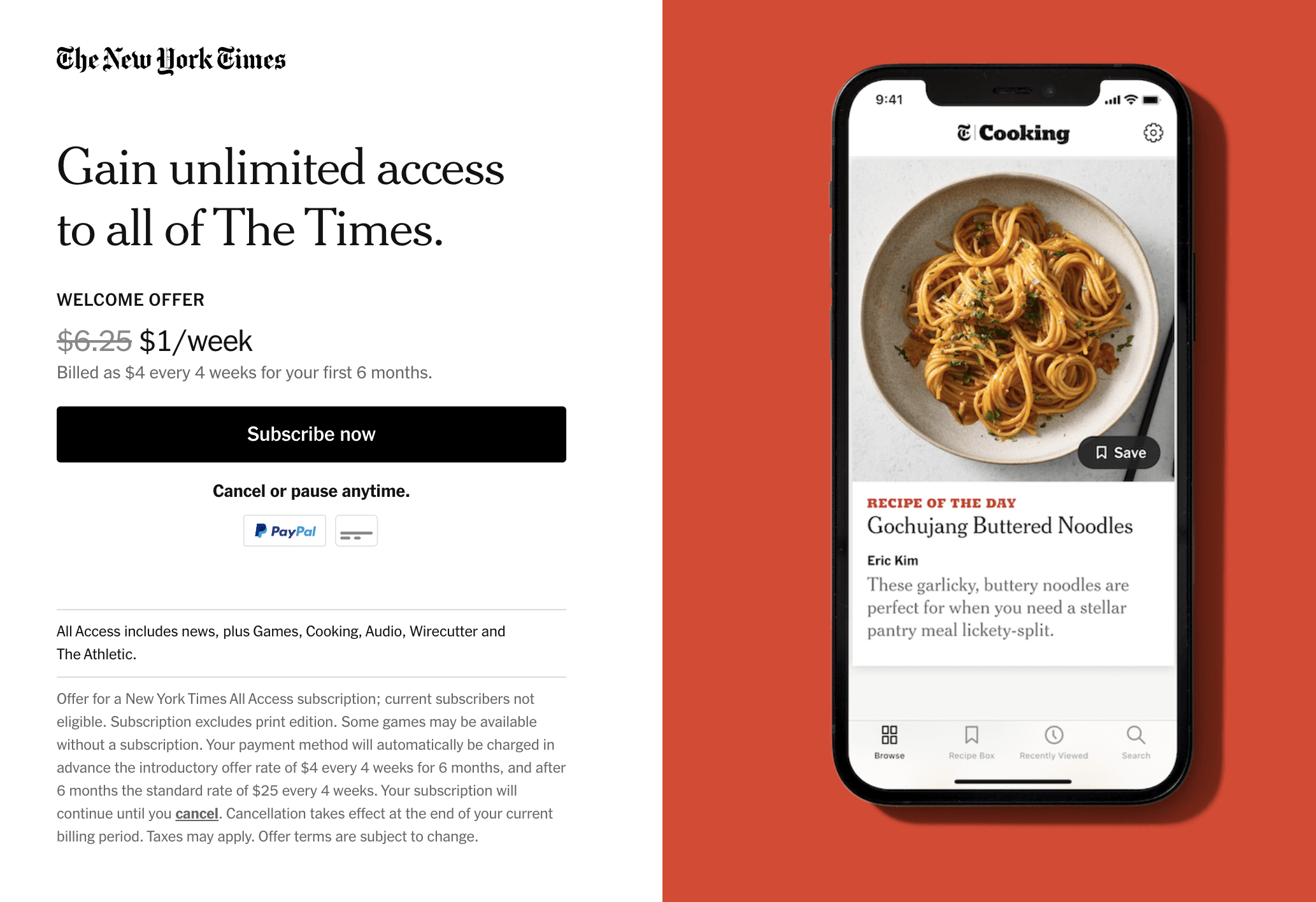The advertisement screenshot consists of two vertical rectangles side by side; one white and one red. 

**Right Side (Red Rectangle):** 
The red rectangle features a graphic of a smartphone lying on the surface, indicated by a subtle shadow to the right of the device. The smartphone has a black bezel and displays a white screen. The screen's content is as follows:
1. The title "Tea Cooking."
2. A section with a plate of spaghetti labeled "Save."
3. The text "Recipe of the Day: Gochujang Buttered Noodles by Eric Kim."
4. A brief description: "These garlickly buttered noodles are perfect for when you need a stellar pantry meal lickety-split."

**Left Side (White Rectangle):**
At the top of the white rectangle, "The New York Times" is written in black font. Below it, a larger black font reads, "Gain unlimited access to all of The Times." Further down, the text "Welcome Offer" is followed by a price of "$6.25" in grey with a line through it. Next to it, the new offer price is displayed as "$1/week," with a note indicating that it is billed as $4 every four weeks for the first six months. Towards the bottom, there is a black rectangle with the text "Subscribe Now" in white font.

This advertisement effectively promotes a subscription offer for unlimited access to The New York Times, appealing to readers with a highlighted recipe feature by Eric Kim.